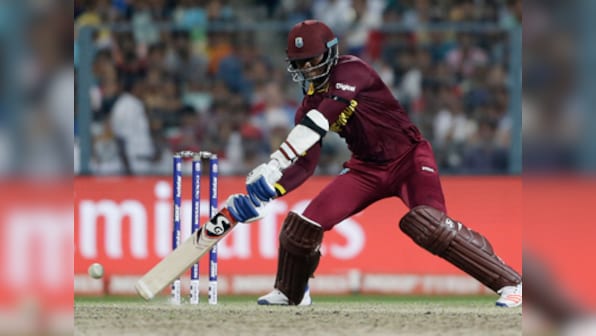This image captures an intense moment during a cricket match. At the center is a player in a maroon uniform consisting of a maroon helmet, jersey, and pants. His protective gear includes brown shin guards extending from his feet to above his knees and arm guards reaching almost to his shoulder. The player stands poised with a rectangular cricket bat, ready to strike a white ball hurtling toward him from the left-hand side of the frame.

In the background, blurred yet slightly discernible, is a crowded stadium filled with enthusiastic fans. Behind the player stands a red half-wall adorned with partially visible white lettering, possibly spelling out "M.I." or "MILARS." Further emphasizing the sporting environment, the ground is covered in green turf, contrasting with the vivid maroon of the player's attire. Blue poles behind the player, resembling a giant "M," add another layer of detail to this dynamic scene.